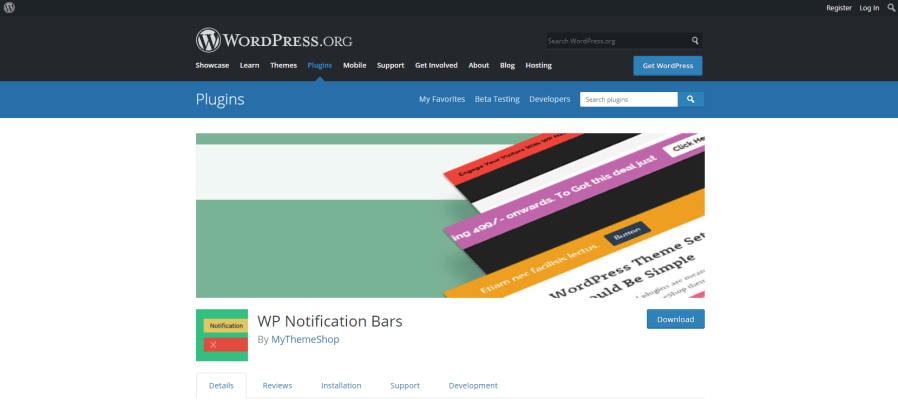This is a detailed screenshot of a WordPress.org webpage. At the very top, there is a large charcoal black bar. In the upper left corner of this bar, there is a logo—a white circle with a black "W" inside it. Adjacent to this logo, text options for "Register" and "Login" are prominently displayed, along with a magnifying glass icon.

In the center of the charcoal bar, the logo appears again, accompanied by the text "wordpress.org." To the right of this, there is a darker black search field featuring the placeholder text "Search wordpress.org" and a white magnifying glass icon.

Directly below the top bar, a site navigation menu is presented in white font. The clickable items in this menu are: "Showcase," "Learn," "Themes," "Plugins" (which is currently selected and highlighted in blue), "Mobile," "Support," "Get Involved," "About," "Blog," and "Hosting." To the right of these menu items, there is a blue rectangle button with the text "Get WordPress" in white.

Below the navigation menu, a blue bar with white font displays additional options: "Plugins," "My Favorites," "Beta Testing," and "Developers." This section also includes a white search field with a blue magnifying glass icon labeled "Search Plugins."

The main content of the webpage is set against a white background. At the top of this section, a graphic showcases three open WordPress pages. Below this graphic, the text "WP Notification Bars by MyThemeShop" is prominently displayed.